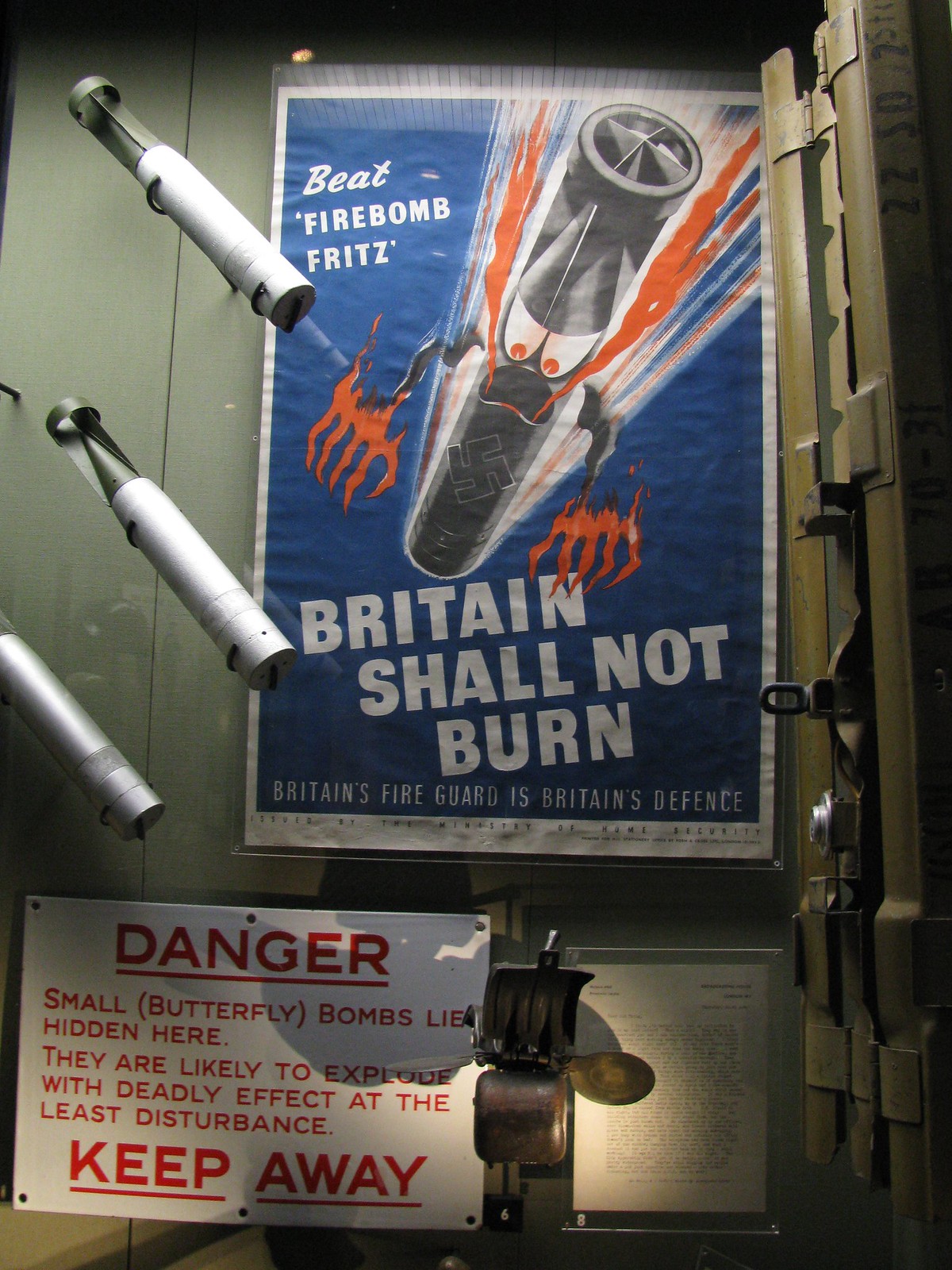This image primarily features a historically-themed propaganda poster with a blue background and prominent white lettering that reads, "Beat Firebomb Fritz." Centrally illustrated on the poster is a cartoon depiction of a menacing firebomb characterized by a cylindrical, elongated body with a Nazi swastika near the base. The bomb has fiery, anthropomorphic features including red, flame-like eyes, a mouth spewing fire, and flame-formed hands suggesting claws. Accompanying the main text on the poster are the emphatic declarations, "Britain shall not burn" and "Britain's fire guard is Britain's defense," both in bold white letters. Surrounding the edges of the poster is a subtle white border.

Below the poster, there's an attached plaque with stark red lettering on a white backdrop that warns, "Danger," followed by smaller text in parentheses, "butterfly bombs lie hidden here, they are likely to explode with deadly effect at the least disturbance," and concludes with a bold, underlined "keep away."

The image also includes a green wall on which the poster is displayed, suggesting a setting that might resemble a museum or an exhibit. To the side of the poster are three suspended models of firebombs, adding a 3D element to the display. The overall ambiance suggests the environment of a bunker or a historically-themed display area.